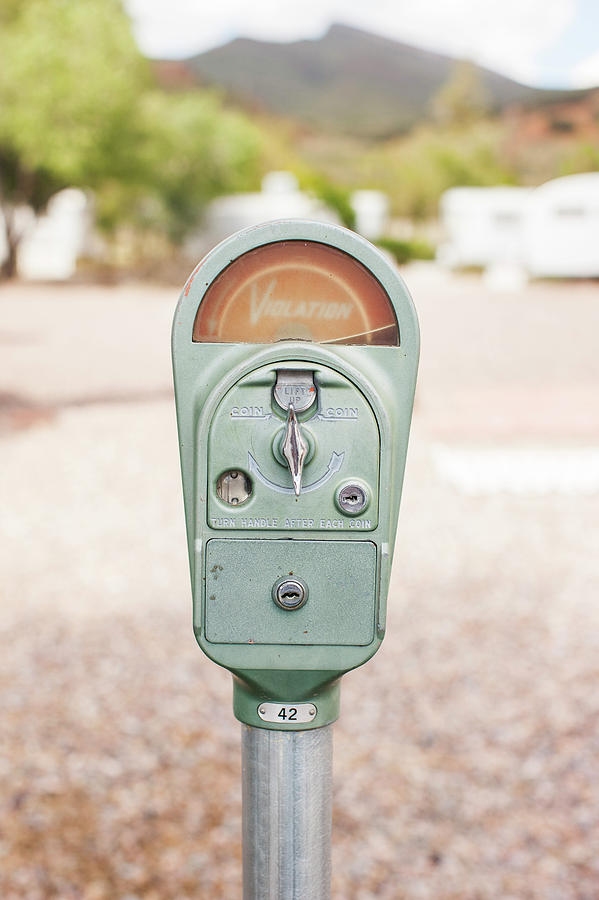In this detailed image taken in portrait orientation, the focal point is an old, classic parking meter standing prominently against a blurred, scenic background. The scene behind the meter includes a dark gray mountain, a soft blue-white sky, and various shades of brown and green from low hills, trees, and shrubs. The indistinct white shapes of RV trailers also dot the background, which rests upon a mottled brown and black speckled pavement.

The parking meter itself features a silver metal pole at its base, transitioning into a teal blue cylinder. Above this cylinder, the meter expands into a vertical rectangle with an arched top and a prominent orange screen that reads "VIOLATION" in white text. Near the base of the teal section, there is a small placard displaying the number "42" in black text against a silver background.

Lower parts of the meter include various operational components: a coin slot labeled "COIN" with an adjacent instruction to "TURN HANDLE AFTER EACH COIN," and an area for inserting and turning keys. A thin, vertical rectangular handle in gray adds to its vintage mechanical charm. Additionally, there are silver colored circles and a lift-up mechanism to access the coin compartment, adding further detail to this well-used piece of urban infrastructure.